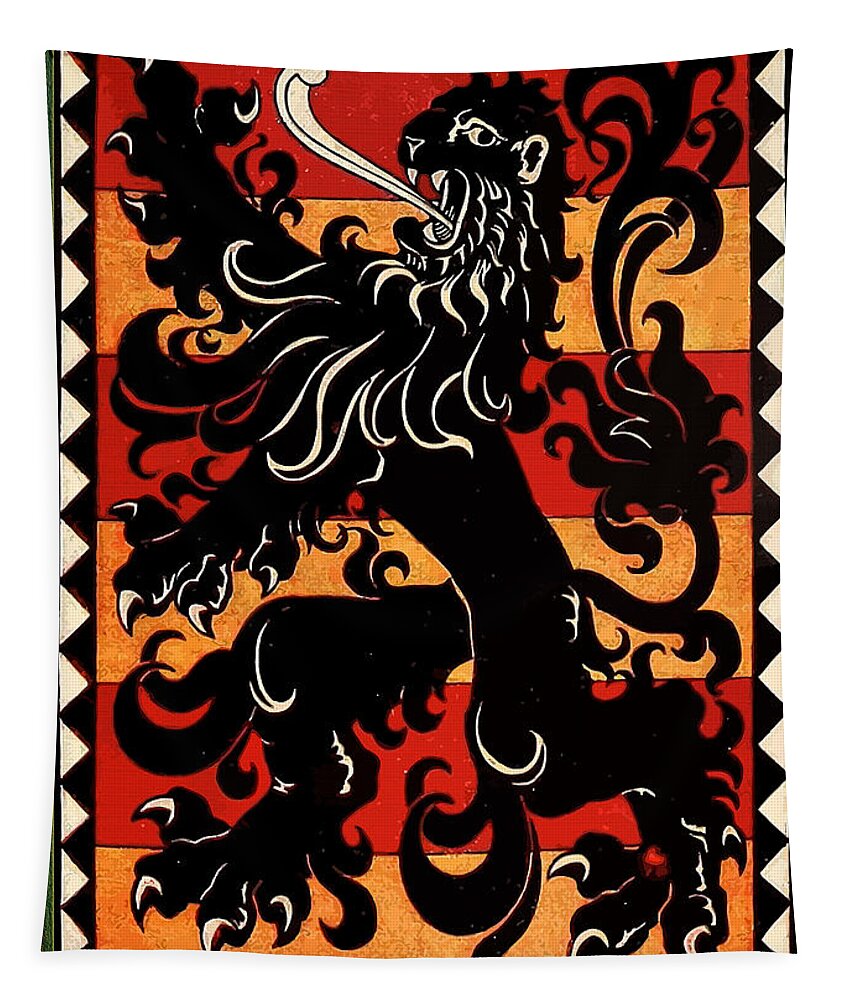This image showcases a vibrant tapestry featuring a central black lion standing upright on its hind legs, facing towards the left. The lion's mouth is open wide, exhaling air, and intricate white highlights accentuate its claws, mane, and teeth. The lion appears to be enveloped in black flames originating from its tail which rise towards the top of the tapestry. The backdrop consists of alternating red and yellow stripes. Along the left and right edges, a black and white triangular pattern extends from the top to the bottom, creating an optical illusion effect. The overall design gives the tapestry a European heraldic appearance.